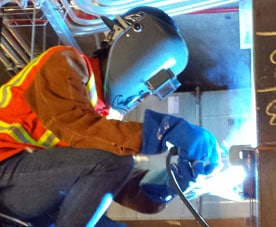The image captures a welder crouching in a small space, performing active welding work. The welder is outfitted in blue safety gloves, a lighter blue welding helmet with a protective glass window, and blue jeans. They are wearing a bright orange shirt beneath an orange and neon yellow safety vest with reflective piping. The intense blue light, smoke, and sparks from the welding process are visible, highlighting the environment. The reflection of the welding can be seen on the welder's helmet. Industrial shelves, various pipes—both metal and plastic—and some white tiling form the background, along with cables or tubes dangling above. The welder holds the welding iron connected to an electrical cable, underscoring the high heat and light involved in their task.